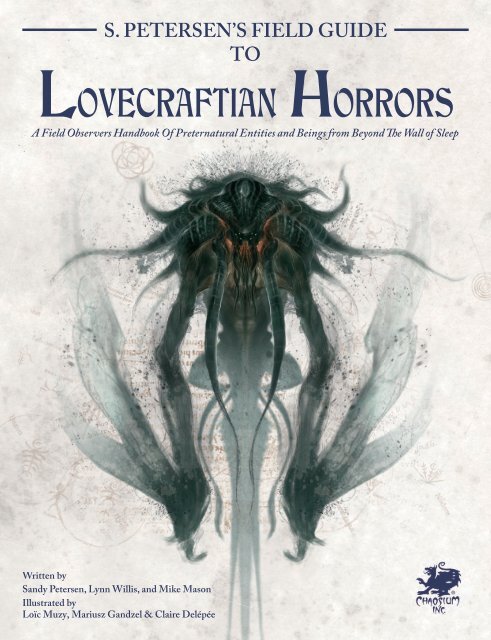The cover of the book "S. Peterson's Field Guide to Lovecraftian Horrors: A Field Observer's Handbook of Preternatural Entities and Beings from Beyond the Wall of Sleep" presents a chilling and mysterious illustration. The creature depicted in the artwork is a nightmarish entity with a distinctly humanoid form, characterized by an ethereal mass of smoky tentacles and tendrils. Its black form contrasts sharply with glowing orange eyes that add to its menacing appearance. The body, vaguely insect-like, has six limbs and emits an aura of otherworldly malevolence. The creature appears both solid and smoke-like, with parts that could be interpreted as drifting wings or vapor, enhancing its alien and preternatural essence. The text at the bottom credits the book's authors—Sandy Peterson, Lynn Willis, and Mike Mason—as well as the illustrators, Loic Muzi, Marosius Gansdell, and Claire Delapee. The cover’s sepia and black-and-white color scheme, combined with the eerie figure, sets a foreboding tone perfect for a guide delving into the realm of Lovecraftian horrors.